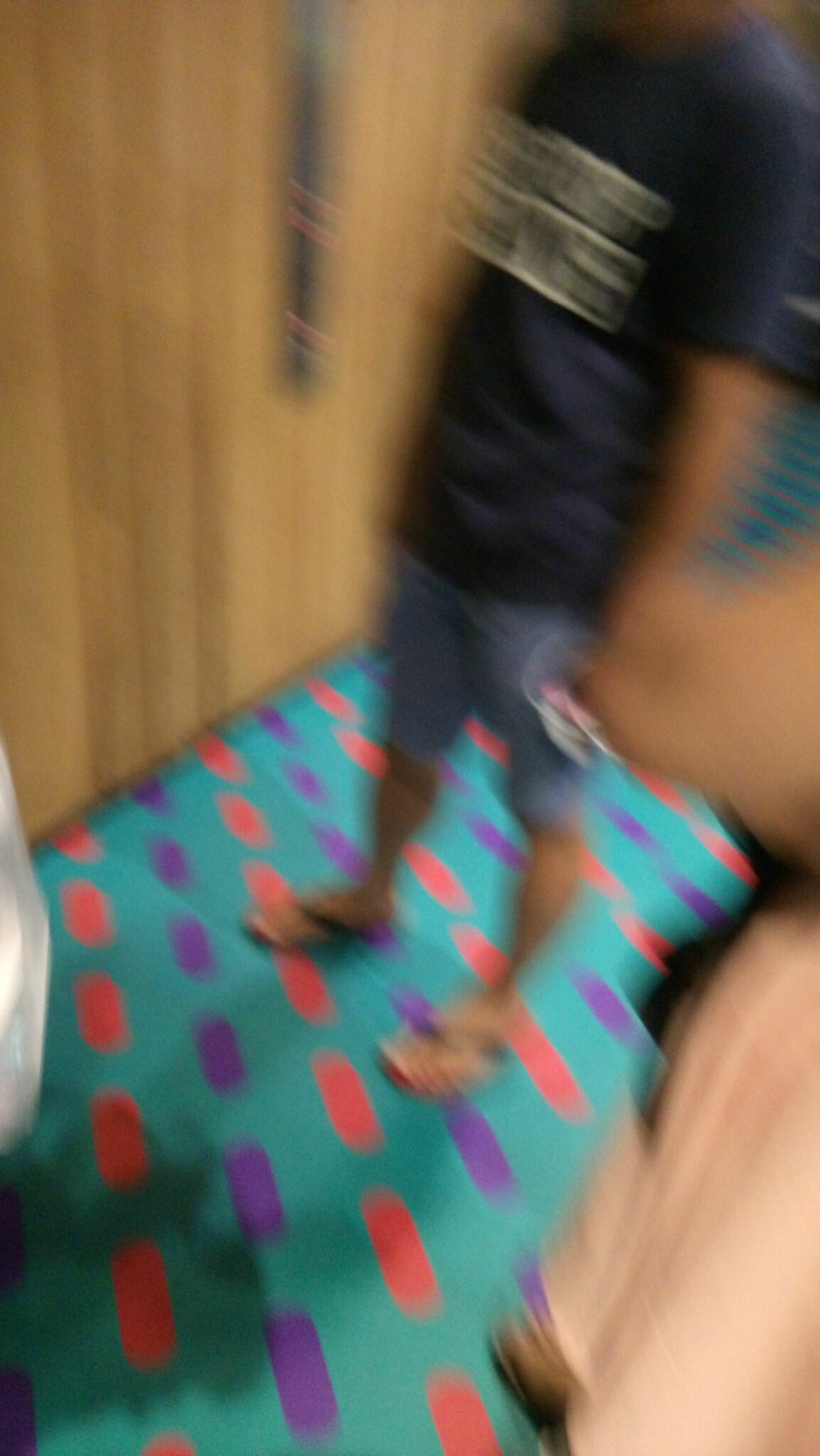The blurry photograph depicts a man standing in front of what appears to be an elevator. The floor features a vibrant turquoise carpet adorned with pill-shaped, oblong designs in colors of purple and pink. The man, who is barely discernible due to the blurriness, wears a navy blue t-shirt with light-colored writing on it, gray or blue knee-length jean shorts, and flip-flops or sandals. Next to him is a brown door, likely with a metal handle. There is also mention of an elevator panel with lit-up lights on the far side of the photo, suggesting the location might indeed be inside an elevator. Another figure, possibly a woman in a flowy pink or peach dress, is vaguely visible, but the lack of clarity makes it difficult to discern any further details. The scene is quite indistinct, but these elements suggest a casually-dressed man waiting with another person in a colorful carpeted setting.